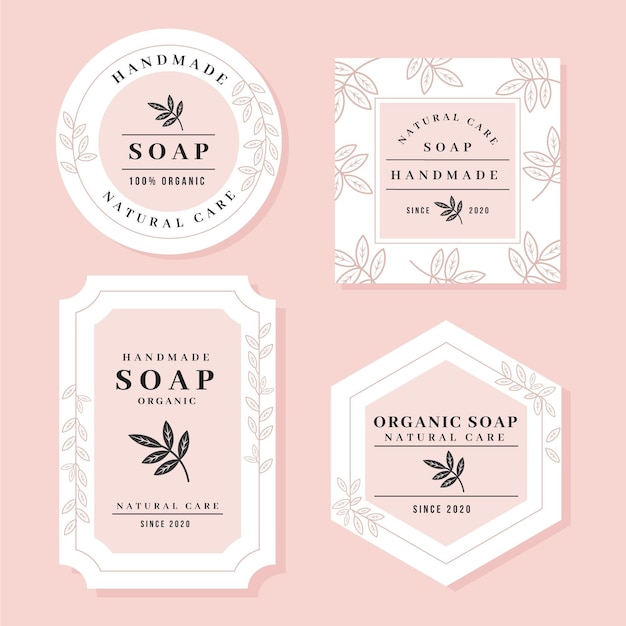This vertical rectangular image features a pink background adorned with labels from four different soap packages, each distinct yet cohesive in design. The labels, centrally positioned against the pink backdrop, incorporate an elegant leaf motif in their design. Each label shares the same core details: "Handmade Natural Care Soap," "100% Organic," and "Since 2020," with text appearing in black or brown.

Starting from the upper left corner, there is a round soap label with a white outer ring and a pink center, showcasing a leaf design and the aforementioned text. To its right, the upper right corner displays a square soap label, also featuring a white border with leaf patterns and a similar pink center with identical text.

In the lower left corner, a rectangular soap label mirrors the design of the previous labels, with white borders and a central pink area carrying the same branding details. Finally, in the lower right corner, a hexagonal soap label completes the quartet, maintaining the consistent design elements: a white border with leaf decorations and the central pink core.

This image effectively functions as an advertisement, highlighting the handcrafted, 100% organic nature of the soaps, unified by the recurring leaf motif, suggesting an emphasis on natural and sustainable care.